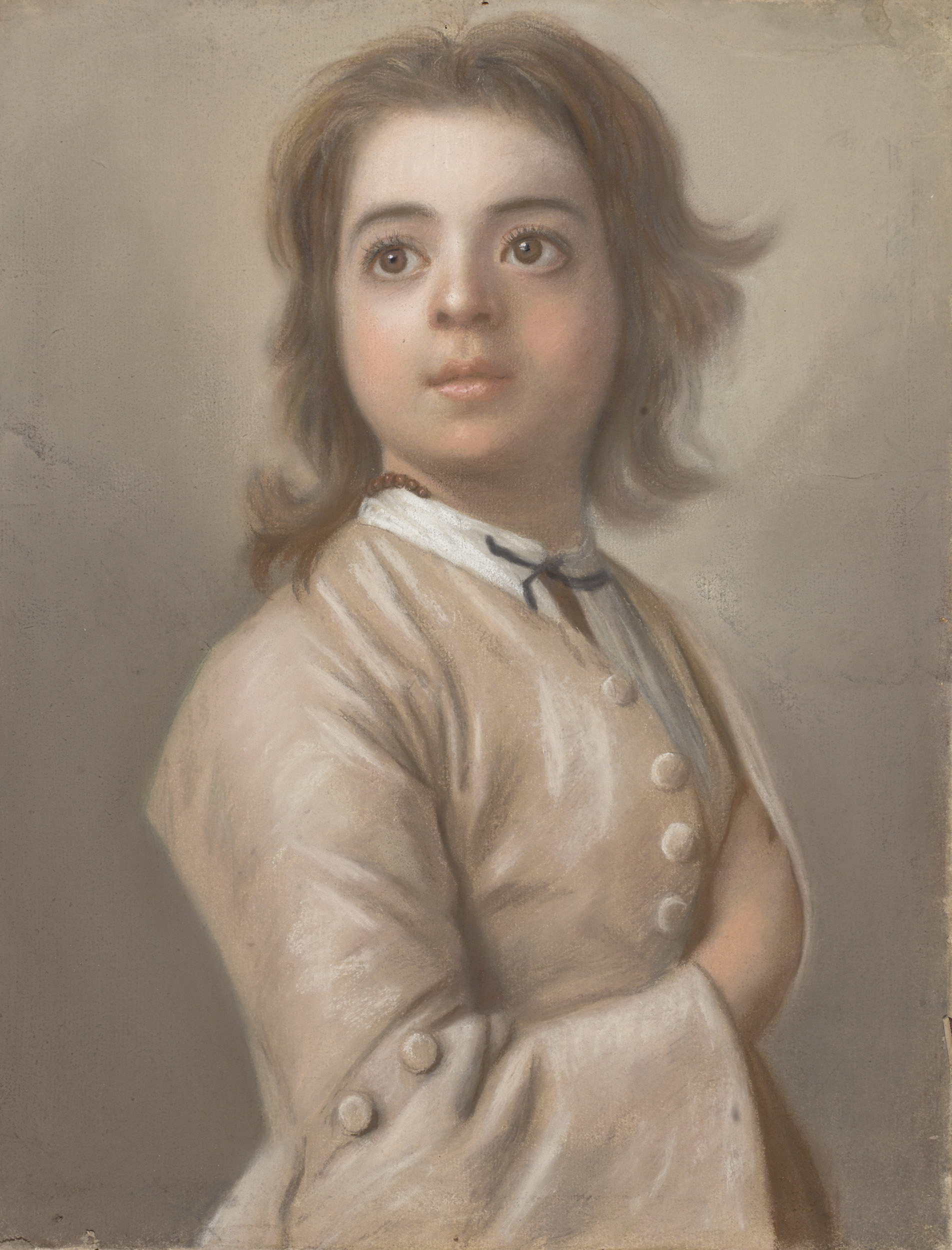The vertically aligned rectangular artwork features a meticulously painted portrait, which appears to be from a few centuries ago, showcasing a young girl who seems to be in her teens. The background is a blend of light and medium brown shades, providing a subtle and timeless backdrop. The girl is depicted with short, slightly wavy brown hair, parted in the middle, and her head is turned towards the viewer while her eyes gaze to the left.

Her facial features include expressive brown eyes, dark eyebrows, and full lips. She is dressed formally in a beige overcoat with long sleeves, which has decorative buttons on the front and additional buttons at the elbows. Underneath the coat, she wears a white blouse paired with a very thin black tie. Positioned inside her jacket lapel, her right hand is bent at the elbow, adding to the formal and composed demeanor of the portrait. The realistic technique captures every detail, from her attire to her slightly unruly yet elegant hair, embodying the essence of historical portraiture with a sense of grace and poise.